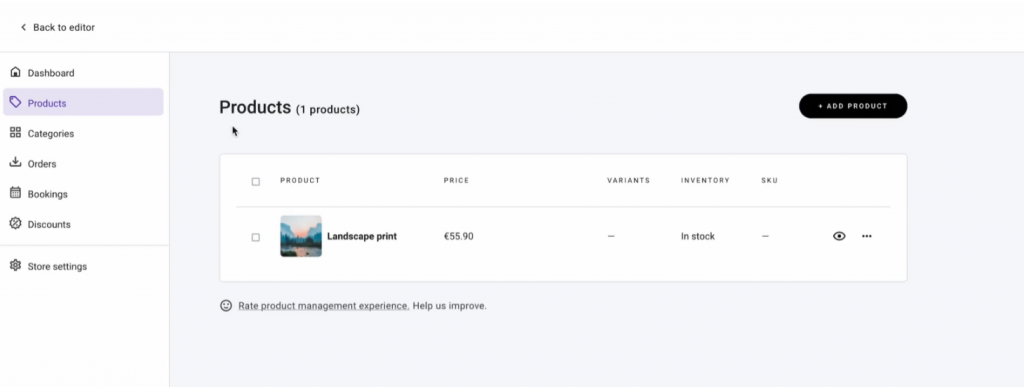This image is a detailed screenshot from a web management interface. At the top left corner of the interface, there is a back arrow icon accompanied by the text "Back to Editor." Below this header, a vertical menu is displayed on the left side, listing various options in black text on a white background. The options include "Dashboard," "Products," "Categories," "Orders," "Bookings," "Discounts," followed by a dividing line, and then "Store Settings." The "Products" option is distinctively highlighted in purple, indicating it is the currently selected section.

The main section of the page displays the heading "Products" followed by a subheading "One Products." Adjacent to this heading, on the right side, there is a prominent black oval button labeled "Add Product." Below this, a table is presented, organizing information with column headers: "Product," "Price," "Variance," "Inventory," and "SKU."

In the first row of the table, there is an image of a painting titled "Landscape Print." The associated details are as follows: the price is listed as "55.90 euros," the variance column is blank, the inventory status indicates "in stock," and the SKU column is also blank. Additionally, there is an eyeball icon button provided to view more details about the product, and to the far right of the row, a three-dot menu offers further actions or options.

At the bottom of the page, an emoji icon accompanied by the text "Rate Product Management Experience, Help Us Improve" invites users to provide feedback about their experience managing products on this page.